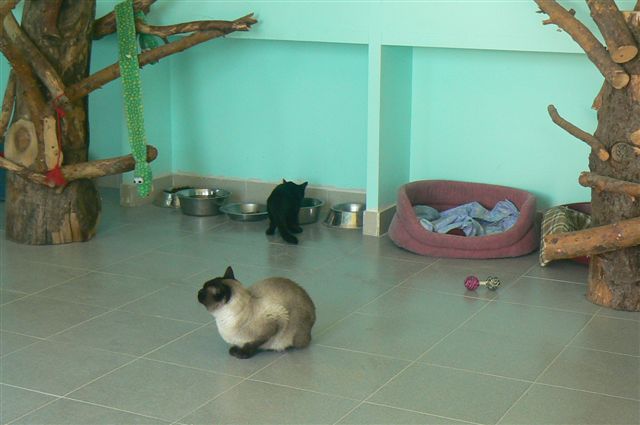This image depicts a cozy indoor scene, possibly a dedicated room for cats or a section of a house like a kitchen. The room has light green walls and a gray tiled floor with a boxed pattern. Dominating the room are two large cat trees positioned in the upper left and upper right corners of the image. The cat tree in the upper left features a long green snake toy hanging from it. 

On the floor, there are five metal cat food bowls lined up, and a black kitten is seen eating from the fourth bowl. In the center of the floor sits a grayish-white cat with black paws and ears, possibly a Siamese cat, curled up in a relaxed bun shape. Nearby, to the right of the bowls, is a fuzzy pink cat bed with a blanket inside.

Additionally, there's a cat toy on the floor consisting of a pink ball connected to a silver ball. This toy, along with other playful cat accessories and the overall setting, suggests a warm and inviting space designed with the comfort and entertainment of the cats in mind.